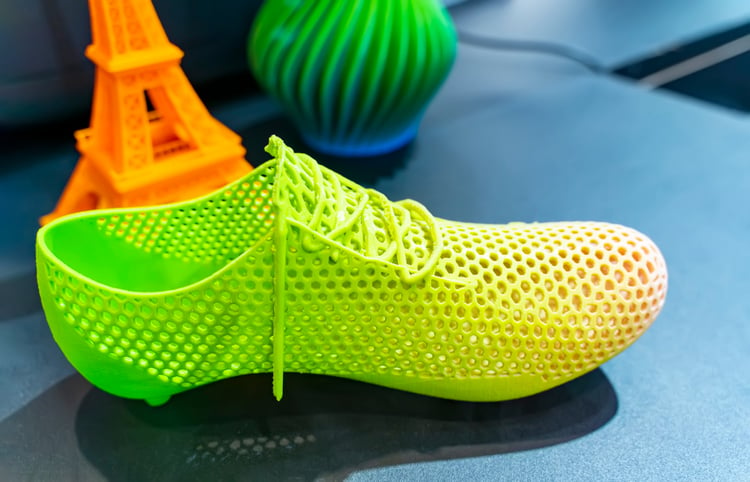On an L-shaped blue countertop, segmented into separate parts, a green plastic shoe with laces is prominently displayed, casting a noticeable shadow. In the background, a white tiled backsplash provides contrast to the scene. To the rear of the shoe sits an orange plastic Eiffel Tower, accompanied by the lower portion of a lime green vase. The vase features a vertically striped pattern in varying shades of green, adding a sense of depth or intricate design. The edge of the counter reveals a white lip, transitioning into a lower blue section.